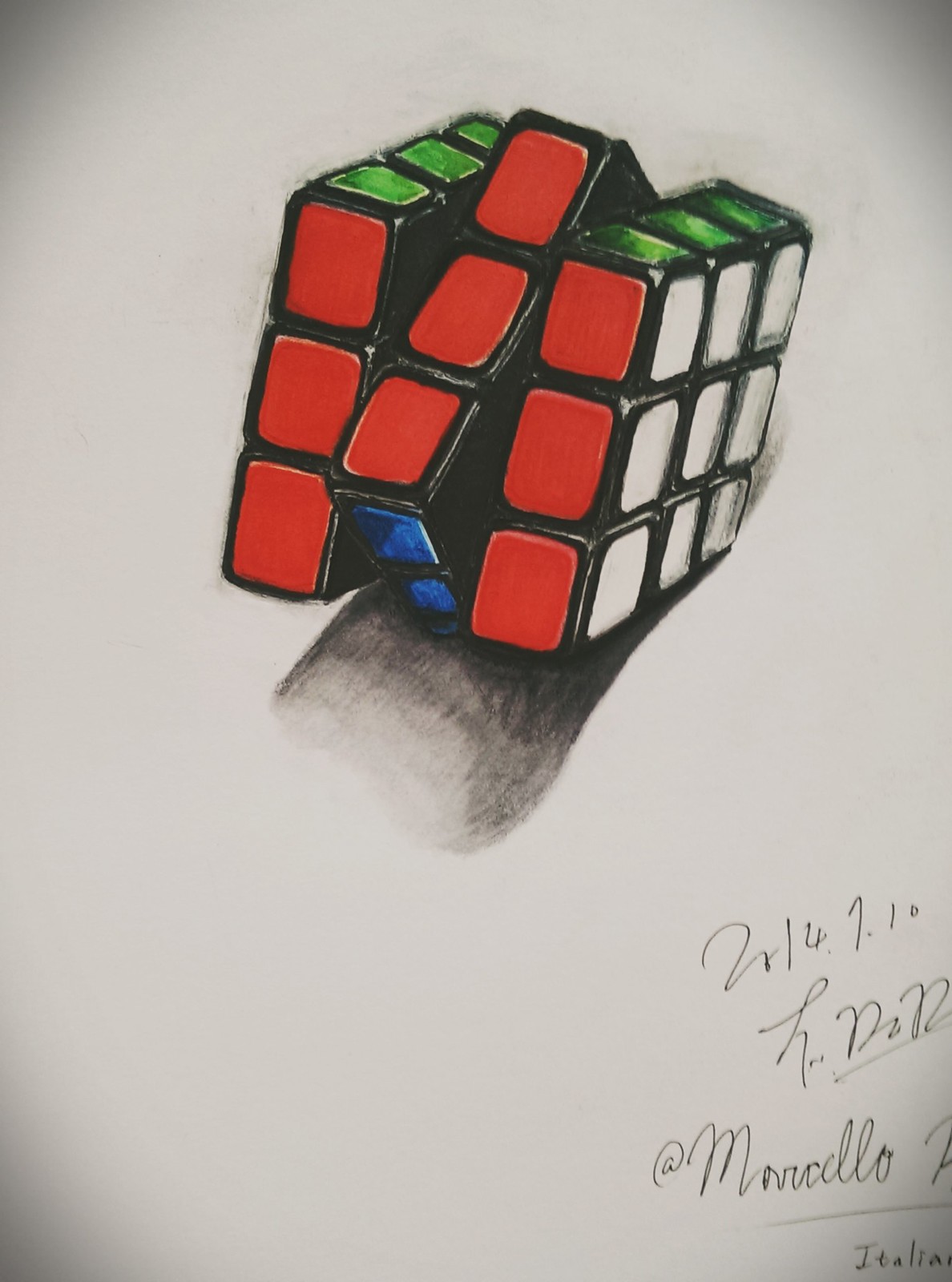This is a detailed photograph capturing a meticulously drawn Rubik's Cube on a white sheet of paper. The cube is presented with the red face prominently displayed at the front, while the right side is composed of nine white squares. The top side of the cube features two visible rows of green squares, and the bottom edge reveals two blue squares, suggesting the twisted orientation of the middle row. This twist causes part of the blue bottom face to become visible, obscuring the top green row. A shadow is rendered beneath the cube using a gray pencil, adding depth and dimension to the illustration. The bottom right corner of the paper bears cursive text written in black ink pen, which reads "at Marcello" with the word "Italian" positioned underneath, indicative of the artist's signature.